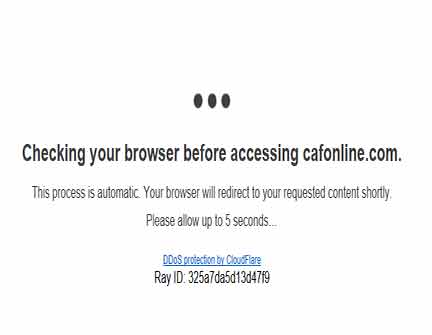This image is a screenshot that typically appears when a website is verifying an individual's request to access its content. The screen displays a moving ellipsis, indicating an ongoing process. At the bottom of the image, a message reads "DDoS protection by Cloudflare," along with a RAID identifier. The primary message on the screen states, "Checking your browser before accessing kafonline.com. This process is automatic. Your browser will redirect to your requested content shortly. Please allow up to five seconds." This verification step is designed to protect the website from Distributed Denial of Service (DDoS) attacks, ensuring that users are legitimate and not attempting to overwhelm the site with malicious traffic. This process is a common and quick security measure, typically taking only a few seconds to complete.